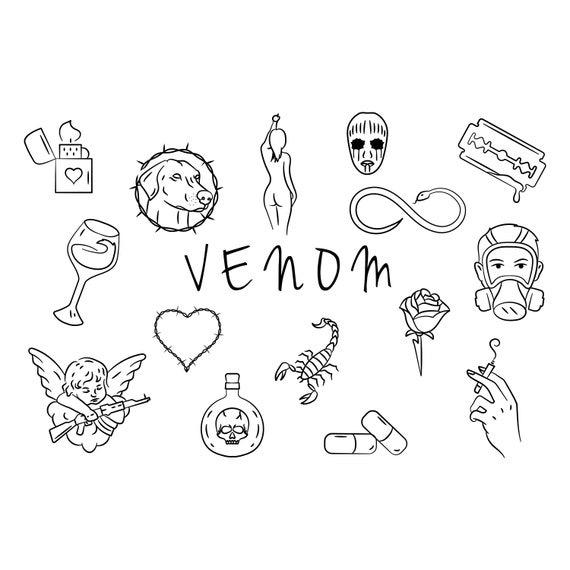This black and white pencil drawing depicts an intricately detailed collage of seemingly random objects surrounding the central word "venom," which is written in a childlike script. Each item is scattered across the white background, meticulously drawn with fine lines and no color filling. Prominently featured are a variety of symbolic elements: a lit lighter with a heart on its casing, a delicate wine glass, and a cherub holding a rifle. Adding to the eclectic mix are a human heart with detailed border lines, a menacing bottle marked with a poison symbol, and a scorpion poised to sting. The illustration also includes a pair of small pills, an elegant rose, and a hand gripping a cigarette. Notably, a figure wearing a gas mask and another, viewed from the back, who appears unclothed, add a touch of surrealism. A dog's head entangled in barbed wire and a razor blade with something dripping off it inject a sense of menace. There's a snake forming an infinity sign and a demon-like face. Each object is small but drawn with great precision, creating a chaotic yet cohesive artistic vision that challenges the viewer’s attention to detail and interpretation.